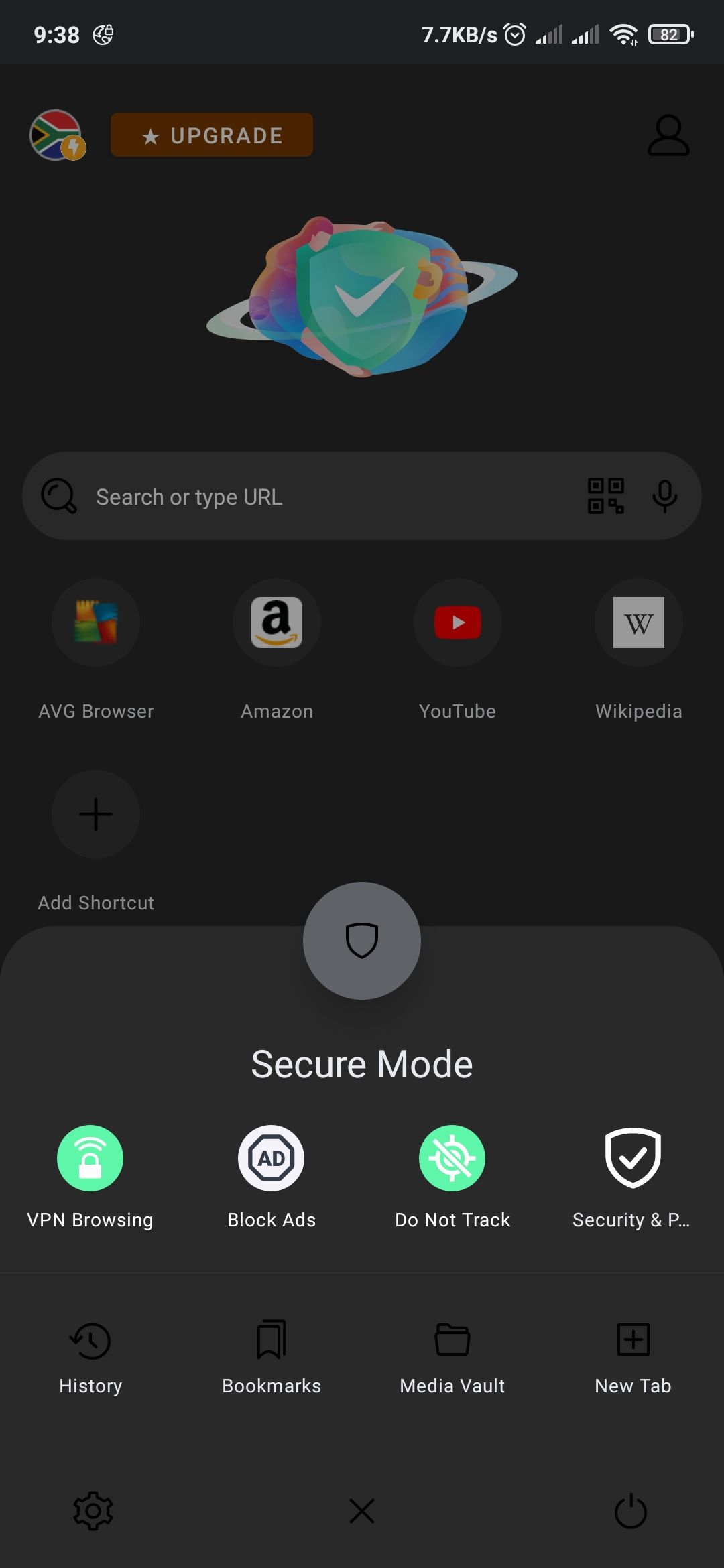The image captures a screenshot of a smartphone in dark mode. The top banner shows a time of 9:38, with no indication of a.m. or p.m. The phone is processing data at 7.7 kilobytes per second and displays an alarm clock icon, signaling that an alarm is set. Additionally, indicators reveal strong Wi-Fi connectivity and a battery level at 82%. The profile icon features a national flag as its picture.

The phone's settings are in dark mode, characterized by the predominance of a black background with minimal white or bright elements. The user has a tab open in a secure browsing mode with various options: VPN browsing is enabled, 'Do Not Track' is selected, but 'Block Ads' is not. A 'Security and Privacy' tab is also present, alongside options for history, bookmarks, and opening a new tab. Frequently visited websites include Amazon, YouTube, and Wikipedia, all accessible from the browsing screen.